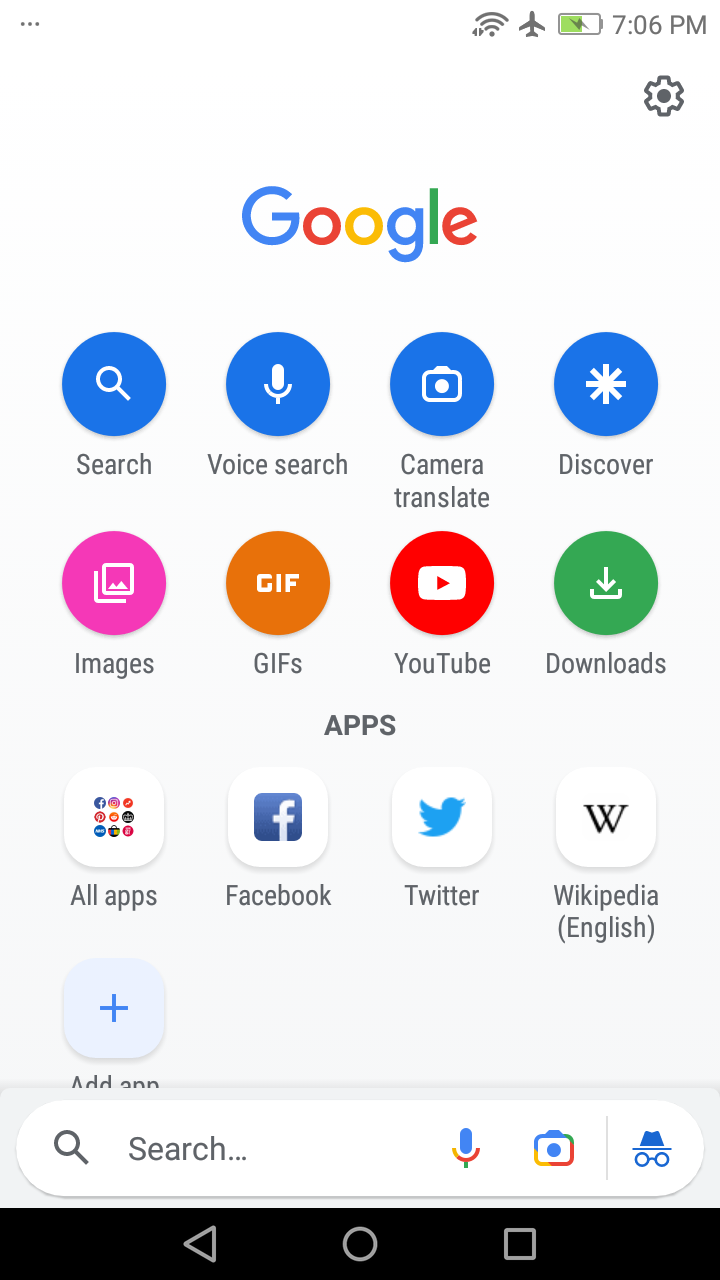The image depicts a Google interface page, starting with the Google logo at the top center. Below the logo, there are various search options illustrated as blue circles: a magnifying glass for standard search, a microphone for voice search, a camera lens labeled "Translate," and a star labeled "Discover." Each icon is matched with an appropriate image to represent its function.

Further down, a row features icons labeled Images, GIFs, YouTube, and Downloads. This is followed by a section titled "Apps," displaying icons for Facebook, Twitter, and Wikipedia, with an option to add more apps. Additionally, at the bottom of the screen, there are icons for a general search, voice search, camera usage, and incognito mode for private browsing.

At the very top of the image, the status bar displays critical information including the current time (7:06), battery life, airplane mode status, and a gear icon for accessing settings. This comprehensive layout represents a standard Google interface, enabling users to search, translate using the camera, browse YouTube, and access downloaded files, all from a single, user-friendly page.